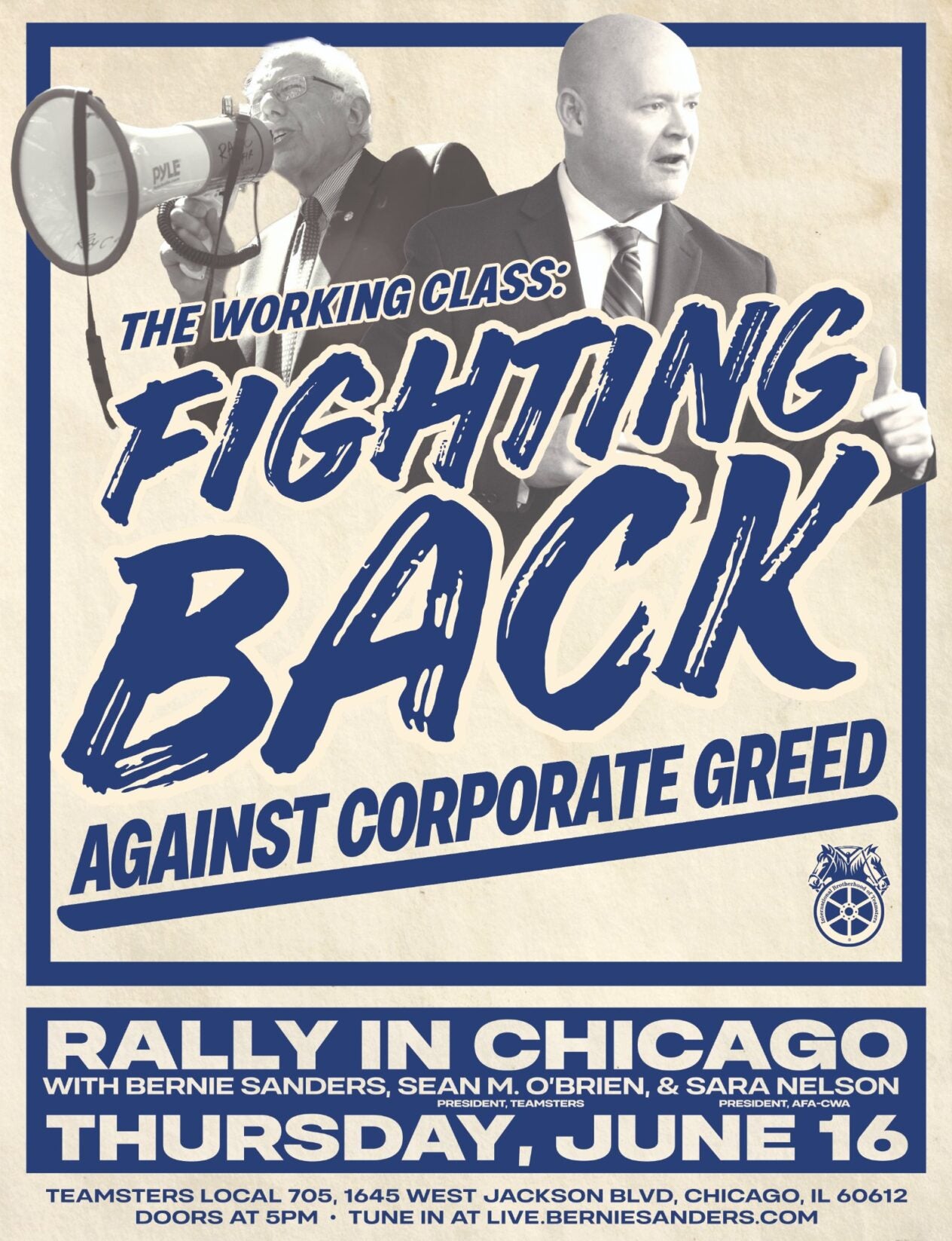This poster features a vertically rectangular multi-color print with an old-fashioned yet contemporary design. It has an off-white outer border followed by a blue inner border, set against a gray paper cardstock background. At the top, there's a black-and-white photograph of a bald gentleman in a suit looking off to the right, with Bernie Sanders in the background to the left, speaking into a megaphone. The central text reads, "The Working Class Fighting Back Against Corporate Greed," with "fighting back" prominently stylized as if hand-drawn with a paintbrush. Below this, in white text on a blue background, the poster announces: "Rally in Chicago with Bernie Sanders, Sean O'Brien, and Sarah Nelson. Thursday, June 16th. Teamsters Local 705, 1645 West Jackson Avenue, Chicago, Illinois. Doors open at 5 PM. Tune in live at BernieSanders.com." This detailed advertisement highlights a political event featuring notable figures Bernie Sanders, Sean O'Brien, and Sarah Nelson.